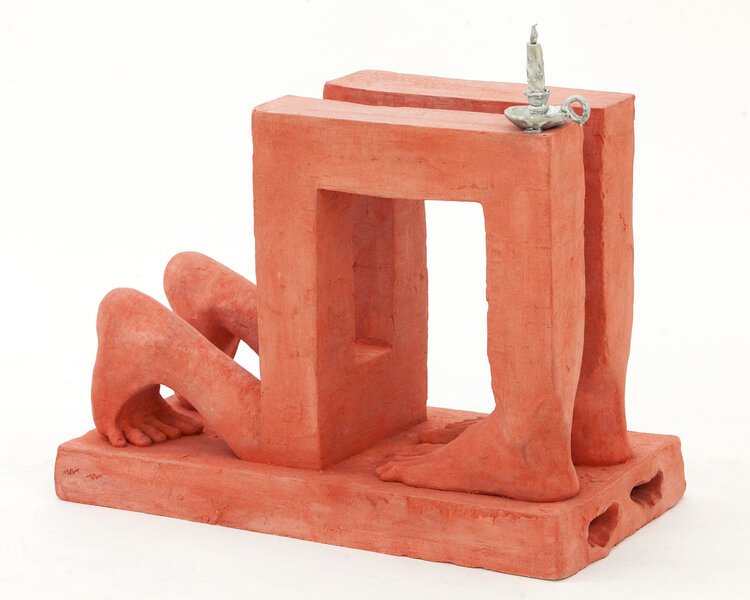The color photograph showcases an abstract sculpture set against a solid grayish background. The artwork, composed of orange clay, features two distinct pairs of human feet. On the right, the feet are standing upright, transitioning from ankles into square, four-by-four fence post-like legs and placed on an orange block base. On the left, another pair of feet are depicted in a kneeling position, with toes resting on the ground and heels elevated. These feet similarly lead into ceramic four-by-four posts that continue vertically and then horizontally, forming a kind of arch. At the very top of the sculpture, a silver candlestick holder with a flame-like element, also made of clay, is prominently displayed. The detailed arrangement and varied shapes create a striking, surreal composition with a focus on the contrasting textures and forms of the feet and the structural elements they evolve into.